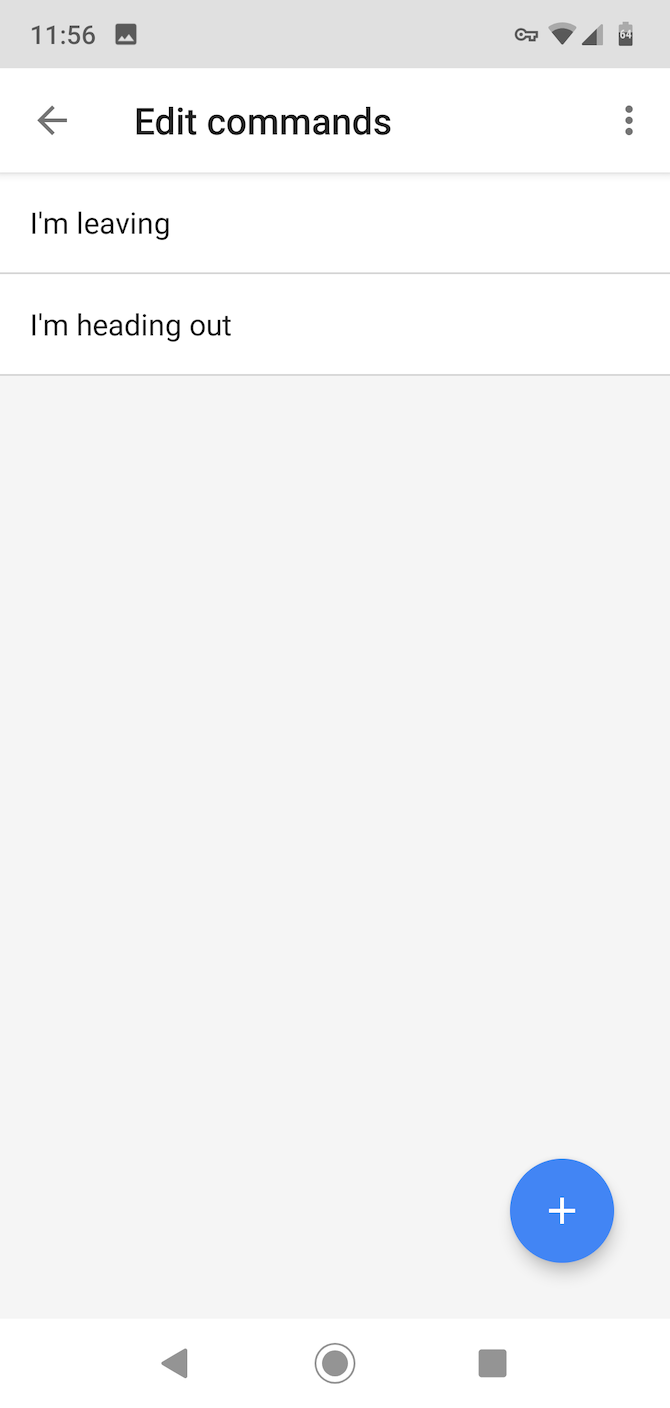This is a detailed screenshot of someone's cell phone screen. 

In the upper left corner, the time reads "11:56," though it does not specify whether it is a.m. or p.m. Moving across the top of the screen to the right, there are several icons: a photo icon, a key icon, a Wi-Fi signal indicator, a cell phone signal indicator, and a battery charge icon showing 64%. 

Directly below these icons, on the left-hand side, there is a left-pointing arrow, presumably serving as a back button. Adjacent to the arrow are the words "Edit Commands" in black letters. Positioned on the far right side next to "Edit Commands" are three vertical dots symbolizing a menu option. 

Below this line of text, there are two statements: “I'm leaving” followed by “I'm heading out.” 

Below this text, there is a large gray rectangular field. In the bottom right corner of this gray field, there is a blue circle with a white plus sign in its center. 

At the very bottom of the screen, there are three navigation icons: a triangle on the left for going back a page, a circle in the center for returning to the home page, and a square on the right for toggling between open apps.